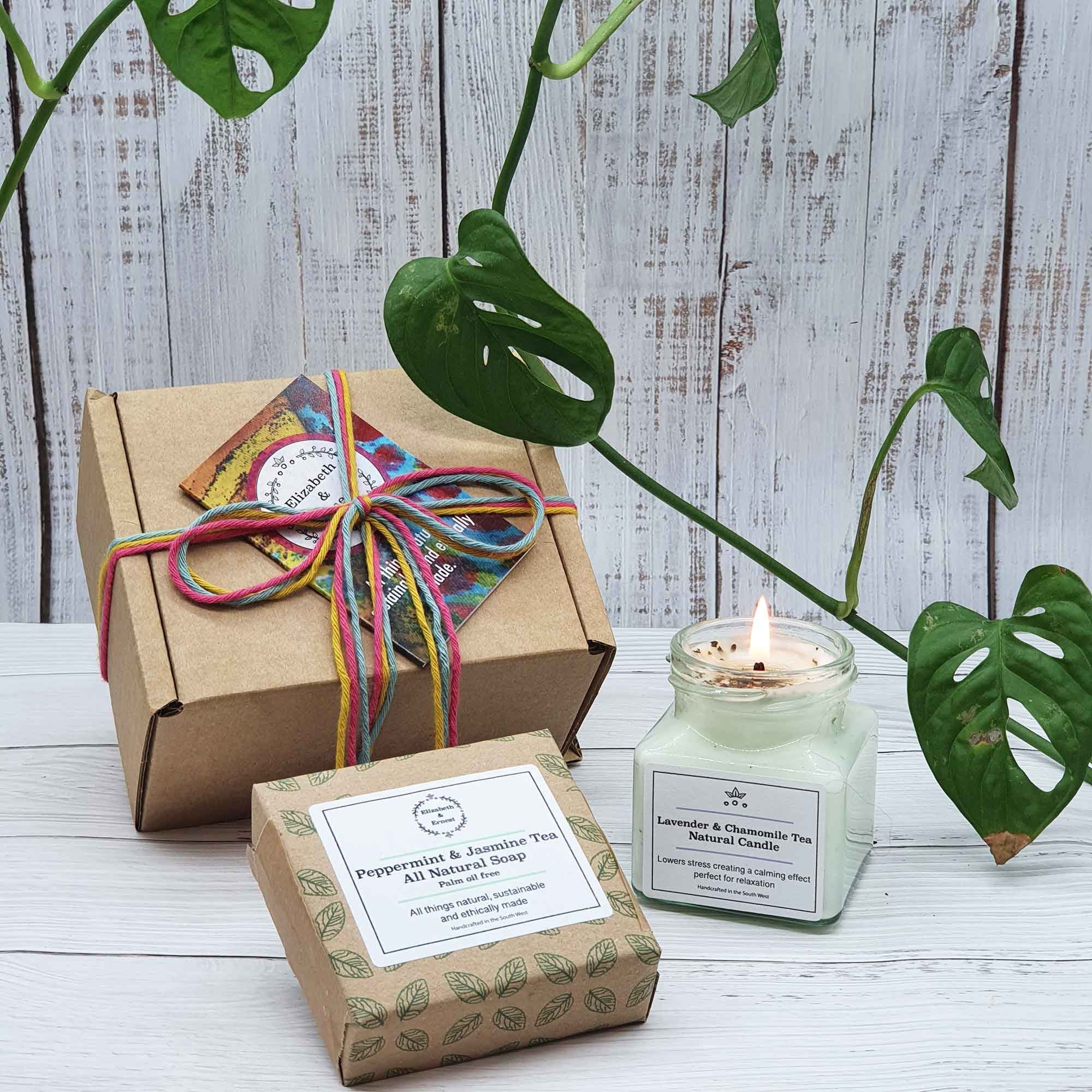This detailed photograph showcases a serene and rustic arrangement on a light gray wooden table, set against the backdrop of a whitewashed wooden fence. A large, wandering green plant extends from the left side of the frame into the center, with various stalks and leaves casting an organic feel across the scene. The table hosts three main items: a large brown box tied with a colorful yarn bow of blue, red, and yellow strings, and adorned with a vibrant pamphlet in hues of yellow, orange, blue, and red. Adjacent to the large box is a smaller brown package wrapped in paper decorated with small green leaves and labeled “Peppermint and Jasmine Tea All Natural Soap” in black lettering on a white sticker. Completing the display, a lit lavender and chamomile tea natural candle, housed in a square glass jar, sits to the right, its soft glow adding warmth. The photograph harmoniously combines elements of nature and handcrafted elegance against the rustic backdrop.